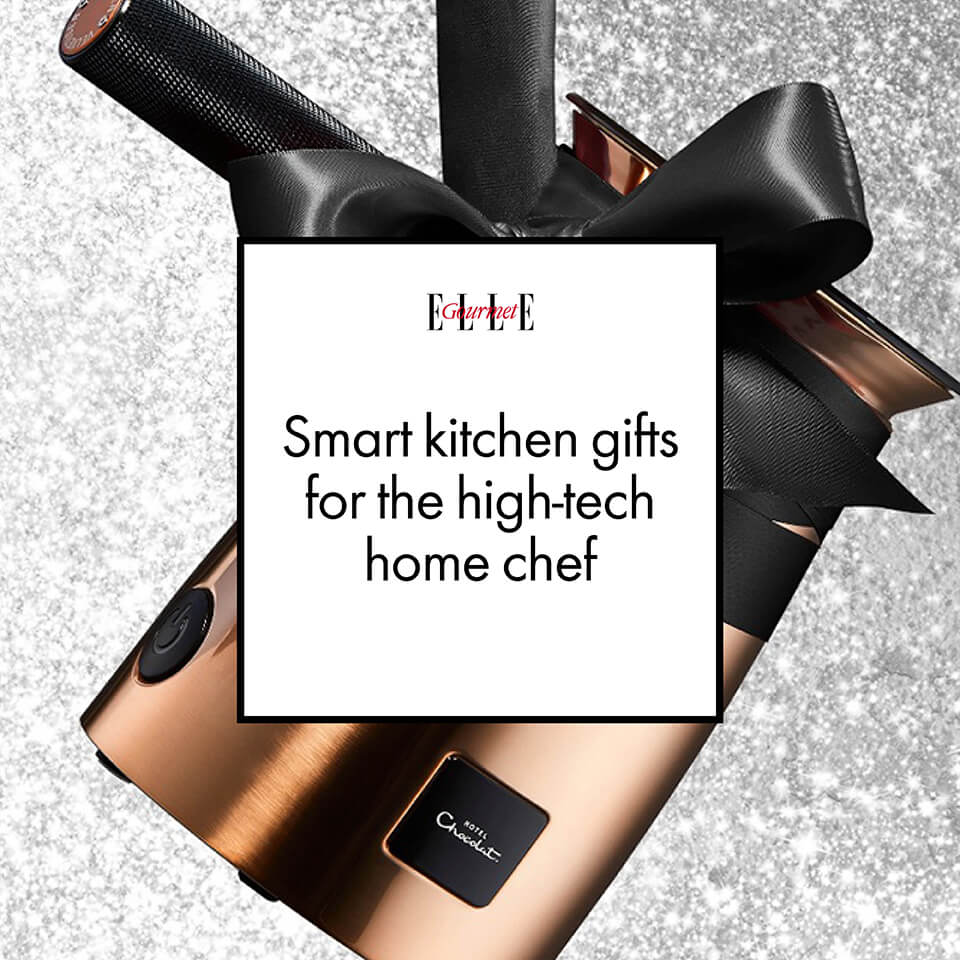In the image, there is a close-up photograph of an electronic kitchen device, wrapped with a black ribbon resembling a bow tie. The device appears to be situated on a gray and white granite countertop. Overlaying the image is a white square watermark with a black border, which partially obscures the device. This watermark contains black text at the top that reads "E-L-L-E" and red text overlaid on that which reads "Gourmet." Below these labels, in black text, it says "Smart Kitchen Gifts for the High Tech Home Chef."

The device itself is bronze or brass-colored with a black power button on the left side and additional black buttons. The top part of the device appears to flip open, revealing more brass detailing underneath and a black handle. The background of the image has a glittery, white, and charcoal pattern that adds a sparkling effect. Overall, the image is an advertisement for "Smart Kitchen Gifts," emphasizing technology and elegance for the modern home chef.